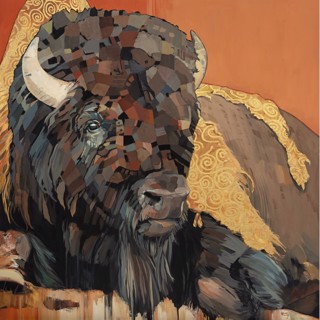This image features an abstract, regal painting of a buffalo, its face presenting a mosaic-like tapestry of varying shades of brown, black, gray, and bluish gray. The buffalo's eyes gaze straight ahead with a sensitive expression, while its distinctive white or tan horns jut out, contributing to its proud demeanor. Below its nose, a mane of long hair accentuates its authoritative presence. Draped over its body is a tan cloth adorned with golden swirls, contrasting with the vibrant orange or red backdrop, adding to the overall majestic and cartoonish style of the piece. The painting emits an almost fantastical aura, blending a multitude of colors and textures for a striking visual impression.